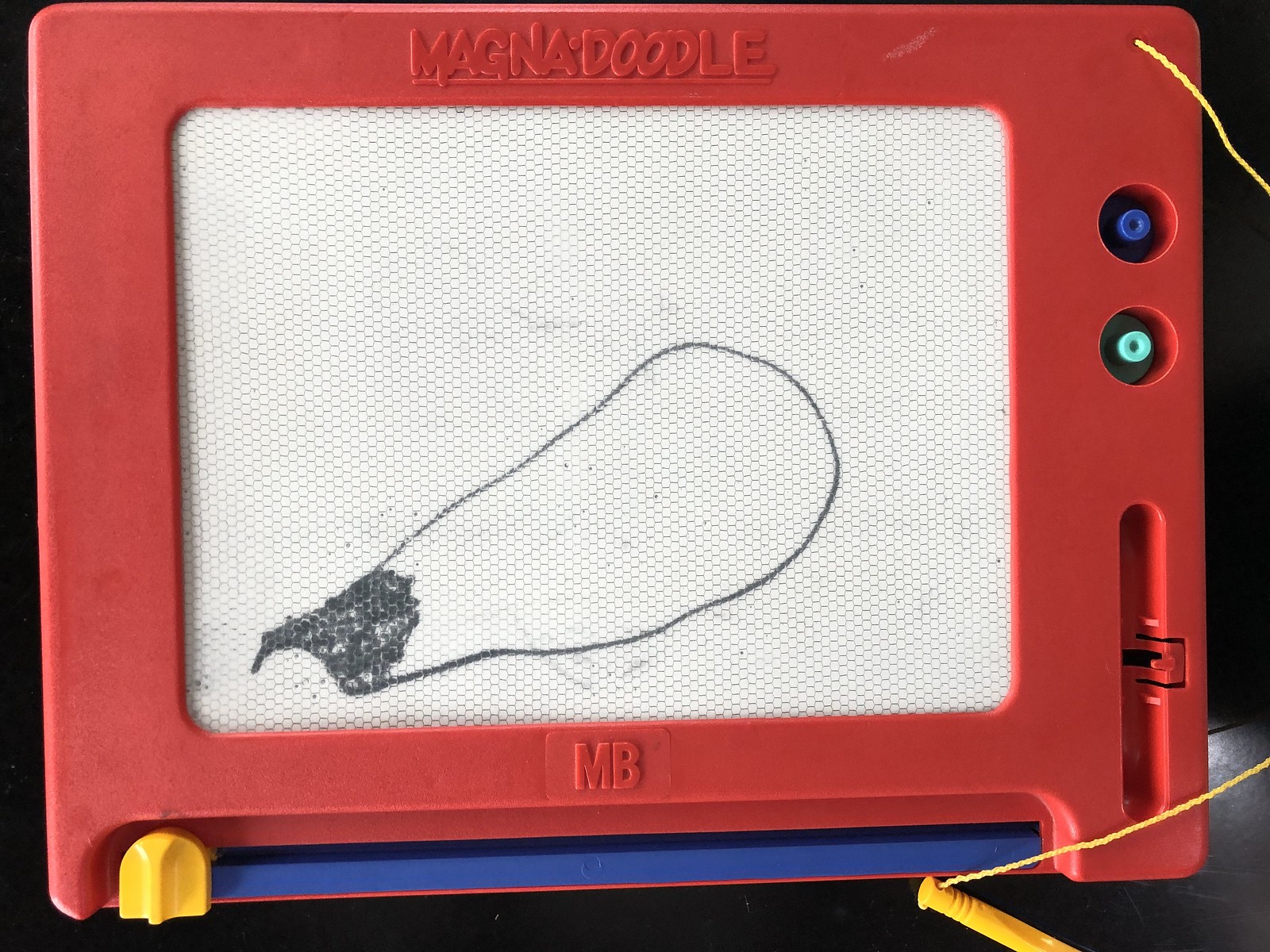This is an image of an unfinished drawing on a red Magnadoodle, with "MB" inscribed at the bottom. The Magnadoodle itself features a vibrant color scheme, incorporating red, blue, yellow, and a turquoise slot for one of the shapes that come with the device. The current drawing on the Magnadoodle appears to be a work in progress, starting from the left and spiraling upwards into a bubble-like form. The initial part of the drawing is notably thicker and shaded, resembling a bride's veil fluttering and about to settle on the ground. This intricate, delicate pattern adds a touch of elegance to the otherwise playful medium.